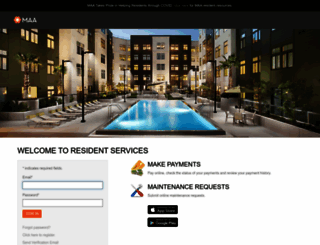A detailed caption for the image could be:

"The image displays a webpage from MAA's 'Welcome to Resident Services' screen, presumed to be part of an apartment rental application where residents can make payments and submit maintenance requests. The page features an option to download the app from both the Apple Store and Google Play Store, along with fields to input an email address and password. The main photo showcases a swimming pool area adorned with lounge chairs on the left side, bordered by several larger residential buildings. Black lamps can be seen encircling the pool area. The MAA logo, featuring an orange sun motif, is prominently displayed at the top, symbolizing the company's branding."